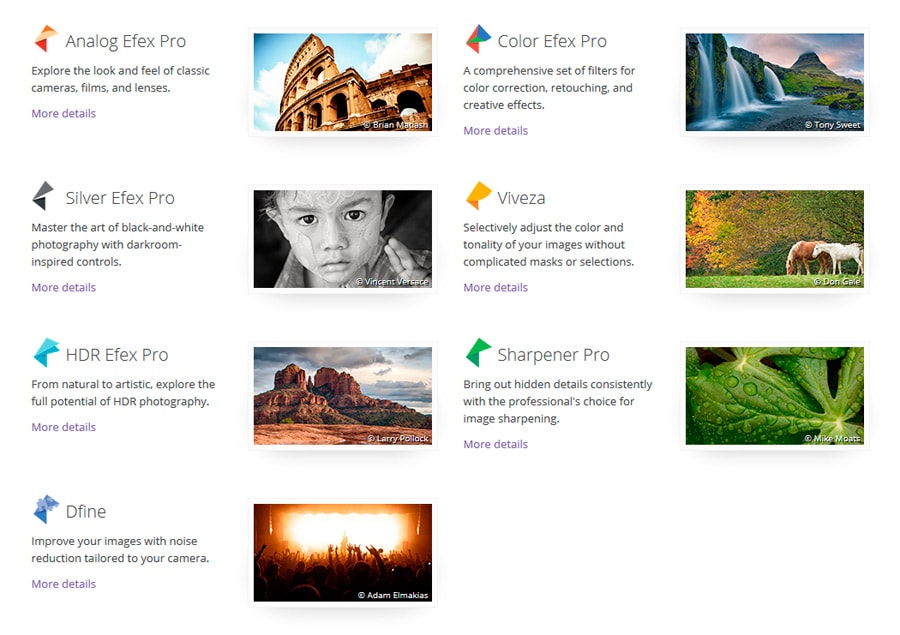This image collage showcases various features of the Analog Effects Pro suite, each represented by distinct, vividly lit visuals:

1. **Silver Effects Pro:** Master the art of black and white photography with darkroom-inspired controls. A striking black and white photo of a child with face paint epitomizes the capabilities of this tool.
2. **HDR Effects Pro:** From natural to artistic, explore the full potential of HDR photography. A dramatic desert mountainscape demonstrates the elevated detail and contrast achievable.
3. **Define:** Enhance your images with noise reduction tailored to your camera. Captured here is a dynamic concert scene, the stage illuminated by pyrotechnics.
4. **Color Effects Pro:** A comprehensive set of filters for color correction, retouching, and creative effects. This section features a lush jungle mountain landscape with waterfalls cascading into a tranquil pond.
5. **Viveza:** Selectively adjust the color and tonality of your images without complicated mask selections. The photograph shows a serene field with horses grazing, colorful trees adorning the background.
6. **Sharpener Pro:** Reveal hidden details consistently with this professional image sharpening tool. A close-up image of water droplets on a leaf highlights its precision and clarity capabilities.

Each segment of the collage serves to illustrate the powerful functionalities and creative potential offered by the suite, making it a versatile tool for photographers and enthusiasts alike.